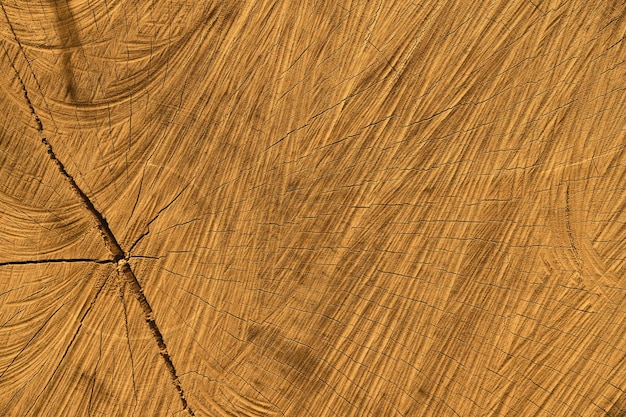This close-up photo captures the intricate details of a sawed tree trunk, revealing its natural wood fibers and organic texture. The surface is characterized by long, sweeping grooves that curve predominantly towards the left side, alongside other curved groove marks on the right. The wood showcases a tannish-brown color, with the tones varying from light brown in some parts to deeper shades elsewhere. A major diagonal crack, starting from the top left and extending towards the middle bottom, dominates the left side, with numerous smaller, natural stress fractures fanning out from this central crevice. These smaller cracks create a complex, web-like pattern interspersed throughout the wood grain. The texture appears rough yet linear, forming both vertical and circular motion patterns that accentuate the natural, untouched beauty of the wood.